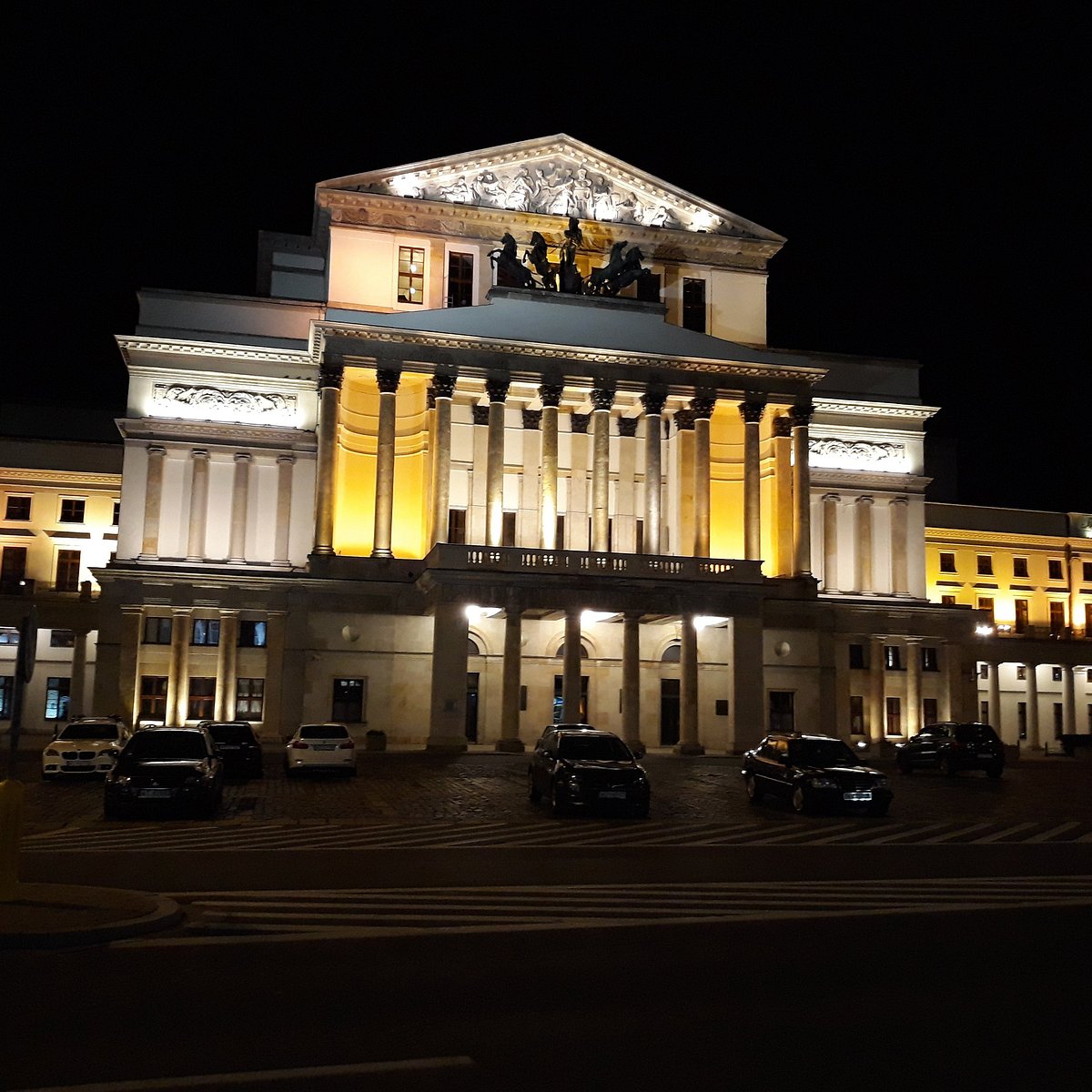This image captures the nighttime view of a grand, historical building, enveloped in darkness with a black sky. The building is beautifully illuminated with a blend of gold and white lights, creating a striking contrast against its beige exterior. The architecture showcases a mix of Greek and Roman influences, with numerous columns adorning both the first and second levels of the facade. The second story features lifelike statues, possibly black statues of horses, while the roof and overhanging sections display intricate carved statues, enhancing its ornate design. The building, which exudes the grandeur of a significant governmental or monumental structure, is accented by the presence of parked cars in the foreground, hinting at its urban location. Despite its familiar architectural style, reminiscent of prestigious buildings found in cities like Washington, D.C., or possibly Florida, its exact identity remains unrecognized.